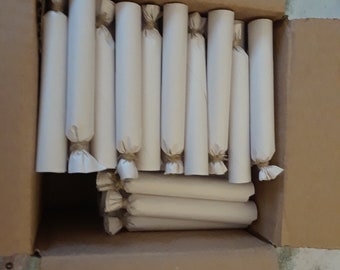This image displays an open cardboard box, brown in color, containing numerous cylindrical items wrapped in light-colored, off-white paper. The paper covering these tubes is tied at the ends with rubber bands or brown strings, resembling a candy wrapper style. The cylinders are stacked both vertically and horizontally within the box. The arrangement creates a varied yet organized pattern, with an empty space noticeable at the bottom left. The box itself is placed on a gray surface, and the open flaps of the box are clearly visible, contributing to the overall rustic and makeshift appearance of the packaging.